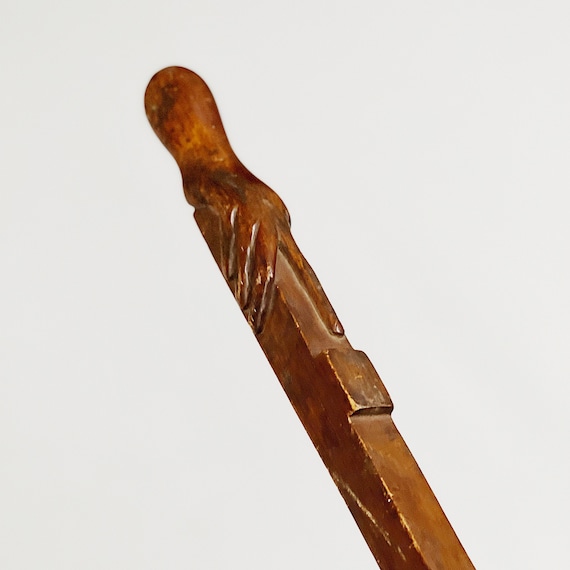This digital photograph features an extreme close-up of a wooden handle, possibly belonging to a cane or walking stick, set against a stark white backdrop. The aged wooden handle is adorned with an intricate carving of a human hand at the top, where the fingers grip the handle and the index finger extends downward along the shaft. The index finger is notably longer than the others, reaching toward a prominent square-shaped groove that juts out from the handle. The handle exhibits multiple scratches and areas where the finish has worn away, particularly around the central square, revealing the lighter wood underneath. The primary colors in the image are shades of brown and hints of gray where the wood has been scratched or rubbed.